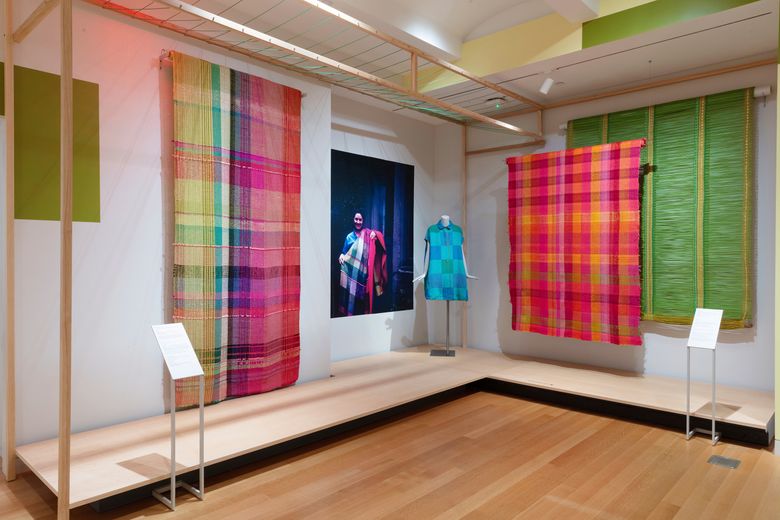The image depicts an exhibit in a textile museum. The room features a hardwood floor that curves gently from the left wall to the right wall, guiding the viewer’s gaze towards a headless mannequin positioned centrally, but slightly towards the far left corner of the image. The mannequin is showcasing a short-sleeved, light blue mini-dress adorned with a checkerboard pattern of darker blue squares. Behind the mannequin, a poster features a woman dressed in a similar checkered shirt.

Along both the left and right walls are large, glass-enclosed structures containing various embroidered and styled fabrics. On the left wall, there is first a green patch followed by a hanging piece of fabric in plaid, with hues transitioning from yellows to greens, blues, and reds. Adjacent to this display is what appears to be a mirror reflecting an image or a picture of a woman wearing a blue and white sari accented with a red scarf.

Moving to the right wall, another piece of plaid fabric is prominently featured with colors in oranges, reds, and some yellow. Behind this plaid fabric is a green material with horizontal threads and vertical yellow stripes, bordered by yellow. Small stands with placards are positioned in front of these glass boxes, providing information about the exhibits. The varied and vibrant array of fabrics, from plaids to embroidered pieces, highlights the intricate craftsmanship and diverse textile traditions being showcased.